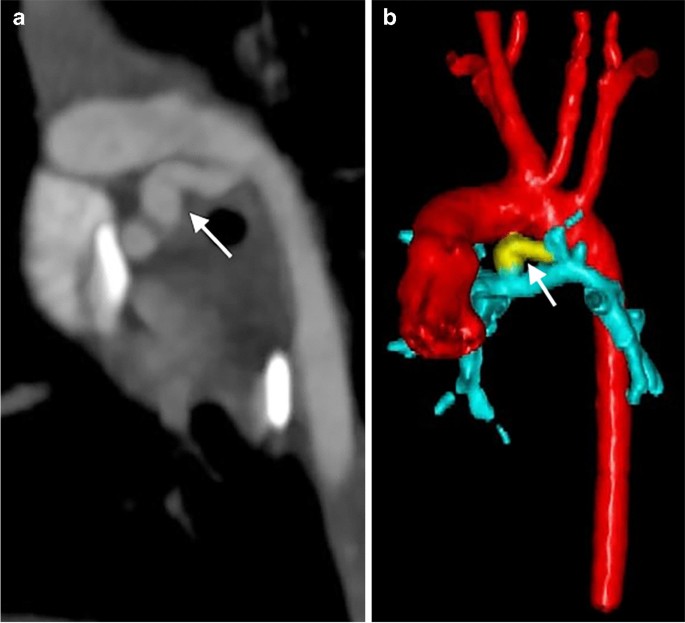The image displays two side-by-side photos of equal height, with the left photo slightly wider than the right. Both images are labeled, with the left featuring a lowercase "a" in the top left corner and the right displaying a white "b" in the same position. The left image appears to be an x-ray or MRI scan, predominantly in light and dark gray tones, focusing on either a stomach or heart area. A cursor arrow in the center points to a distinguishing curved shape.

The right image serves as a 3D-rendered or computer-simulated counterpart to the left image, offering more clarity on the anatomical focus. This image is more colorful, featuring prominent red tubing, likely representing veins or arteries, extending downwards. Additionally, turquoise tubing is also visible. Centrally, a yellow section is highlighted with a cursor arrow, identical in shape to the highlighted area in the x-ray or MRI. This part is positioned between the red and turquoise sections, providing a clearer spatial understanding of the area of interest within the body. Both images are set against a black background, adding contrast to the detailed anatomical features.